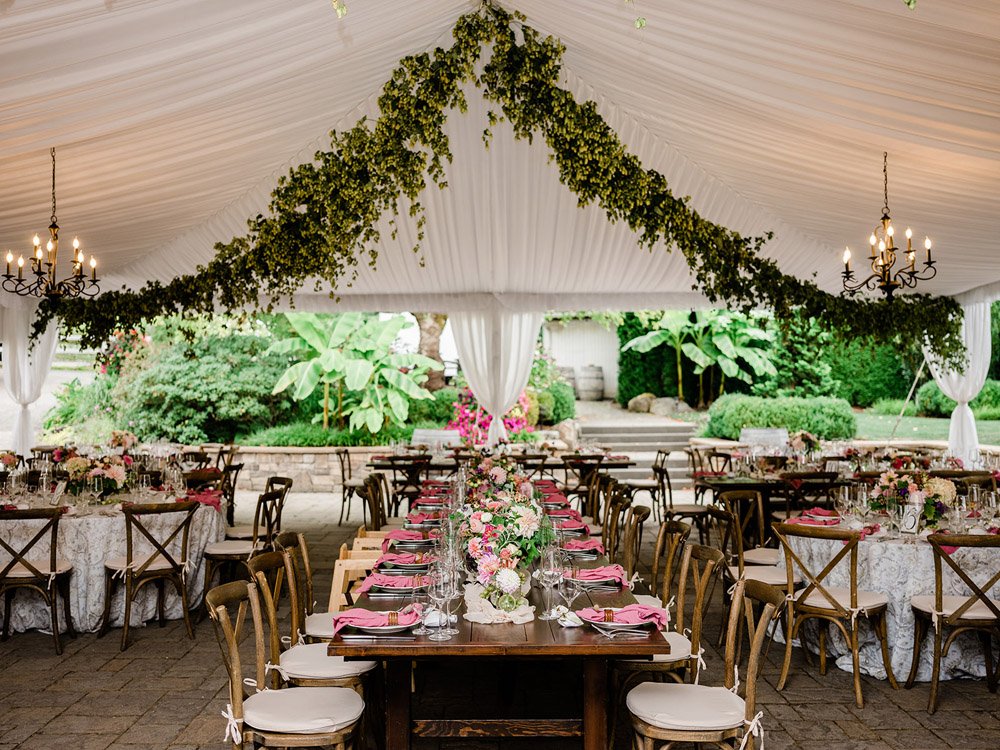This image captures the elegantly decorated setup of an outdoor wedding reception, held under a large, white tent with high ceilings adorned with green ivy garlands and two chandeliers featuring flame-shaped light bulbs. The scene is empty of guests, showcasing a pristine and inviting atmosphere ready for celebration. 

In the foreground, round tables draped in white lace tablecloths are arranged to accommodate ten to twelve guests each. Each table is meticulously set with white plates, bright pink napkins secured with gold rings, glass stemware, and cutlery. The chairs accompanying these tables are wooden with open backs and light tan cushions, adding a rustic touch.

A prominent, long rectangular table sits at the center of the arrangement, lined with similarly set place settings and seating about seven to eight guests on each side. On the left side of the image, darker and wider chairs surround a table featuring a tablecloth, abundant flowers, and additional glassware, contrasted by another table similarly adorned on the right.

The backdrop of the scene reveals an array of tropical plants, bushes, and a lush green lawn, enhancing the natural and vibrant ambiance of the venue. The combination of greenery, elegant decor, and sophisticated table settings paints a picture of an inviting yet opulent celebration space, perfectly staged for a memorable wedding event.